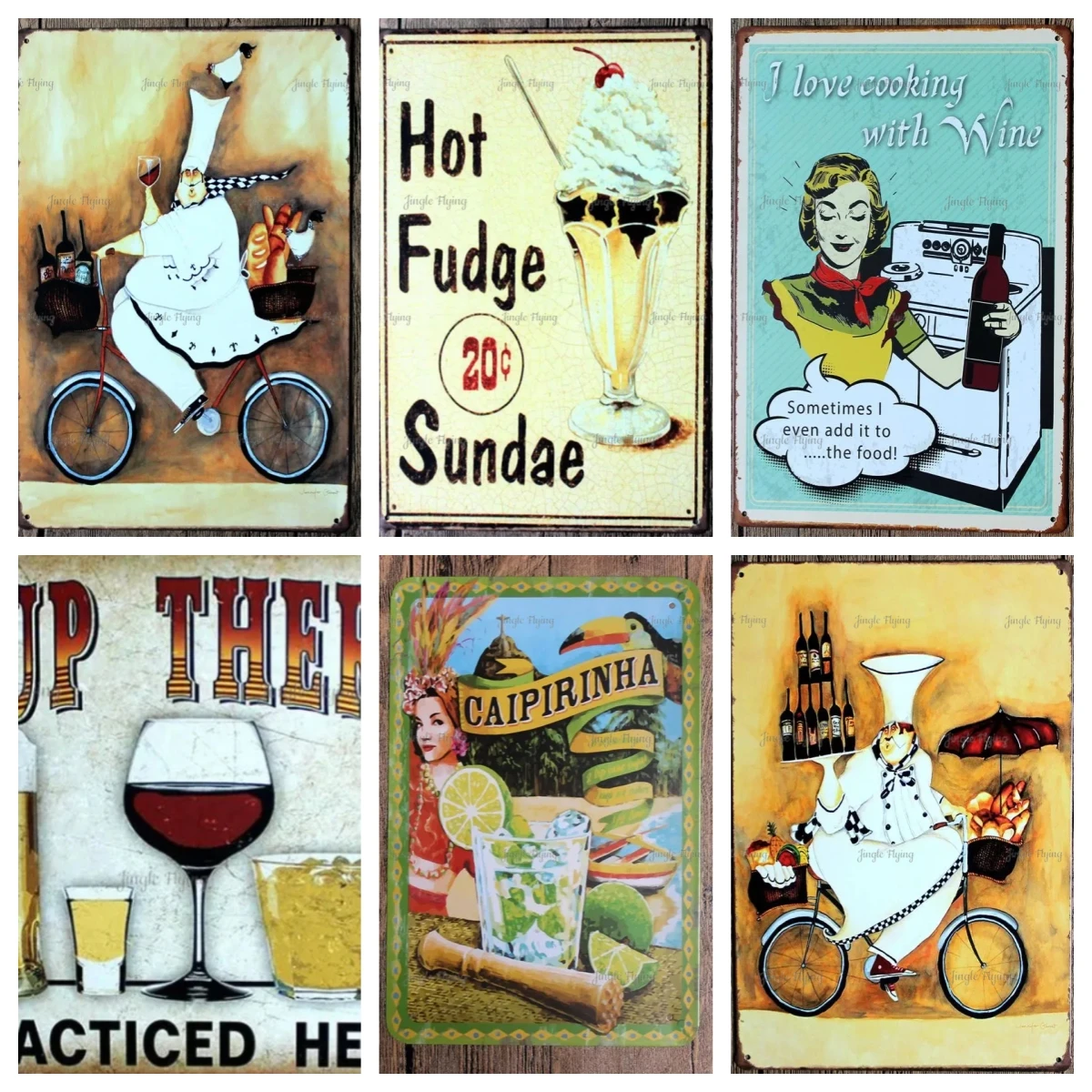This is a collage of six vintage tin wall signs mounted on wooden walls, arranged in two rows of three images each, separated by thin white lines. The top left sign features a jolly, large chef riding a bicycle with a basket of wine bottles in front and bread loaves behind. The top middle sign showcases a hot fudge sundae with the text "Hot fudge sundae 20 cents." The top right sign depicts a retro-styled blonde woman in a yellow apron holding a wine bottle, standing in front of a stove, with the text, "I love cooking with wine. Sometimes I even add it to the food." The bottom left sign is cropped but includes illustrations of a shot glass, a wine glass, and a larger glass, possibly for scotch, with partial, unreadable text. The bottom middle sign shows a tropical-themed beverage with a lime garnish, a toucan in the background, and a woman in a red dress beside it, accompanied by the text "Caipirinha." The bottom right sign is a variant of the top left, depicting the same cheerful chef cycling, this time holding a tray of stacked wine glasses, with a basket of fruits behind.